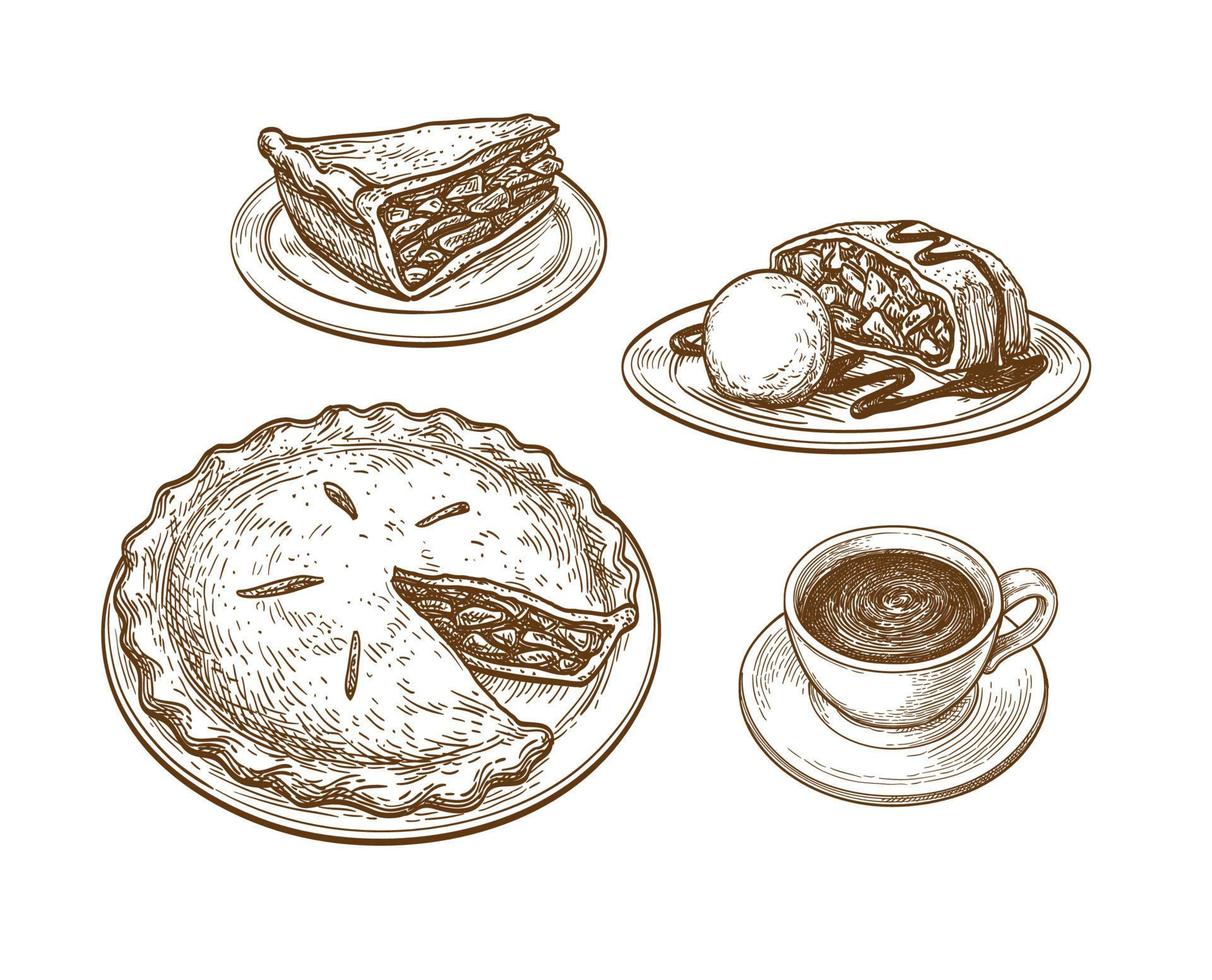This image showcases four brown-toned ink drawings of various desserts on a plain white background. In the bottom left corner, there is a round plate holding a whole pie with a slice missing. The pie, featuring four ventilation slits cut into its crust, seems to be an apple pie with elongated bits of apple visible inside. Directly above, the missing slice is depicted on a smaller plate, matching the pie below. To the right of the whole pie, there is a cup filled with a dark liquid, likely coffee, resting on a saucer. In the top right corner of the image, there's an intriguing dish resembling a crustless pie topped with a dripping dark brown sauce, possibly chocolate syrup, accompanied by a ball-like shape that looks like a scoop of ice cream.